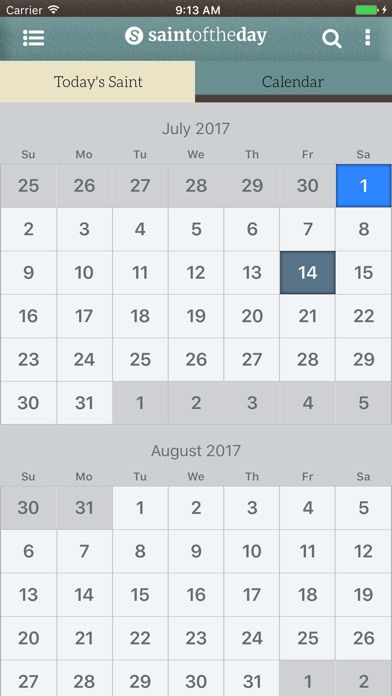The image displays a detailed digital screen interface, resembling a calendar app. In the center-top of the image, the current time is prominently shown as 9:13 a.m. To the right, there is an icon indicating a fully charged green cell phone battery. Next to this, a white circular icon with an "S" in its center is labeled "Saint of the Day," accompanied by a magnifying glass icon for search functionality.

Below this toolbar, the main calendar display starts. The top portion features a beige-highlighted area with the word "Calendar" over a green background, indicating the month of July 2017. The calendar grid itself begins with Sunday, June 25th, and the top row ends with Saturday, July 1st, which is highlighted in a blue box. Subsequent dates continue throughout July, with the 14th of July distinctly marked in a dark green box, while the rest of the dates are in gray boxes.

As the calendar transitions into August 2017, the background color shifts to light gray. Here, the dates continue, starting with Tuesday, August 1st, and concluding on Thursday, August 31st. In the very bottom corner, the numbers "1" and "2" suggest the beginning of September, even though the month of September itself is not displayed in the image.